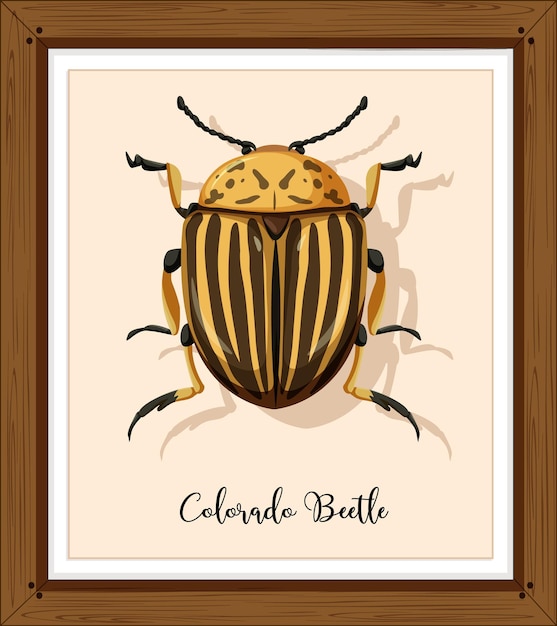A detailed illustration of a Colorado beetle is presented on a piece of pink paper, encased in a brown frame with a white inner border. The beetle, prominently positioned, is a plump and rounded insect. Its body exhibits a light brown coloration accented with several dark brown stripes. The beetle's legs are segmented, featuring black at the top, transitioning to light brown, and ending in black at the bottom. The beetle's back is predominantly light brown, adorned with subtle darker brown markings. Its small black eyes and two protruding black antennae add to the detailed depiction. At the bottom of the image, "Colorado Beetle" is inscribed in black letters, identifying the subject.